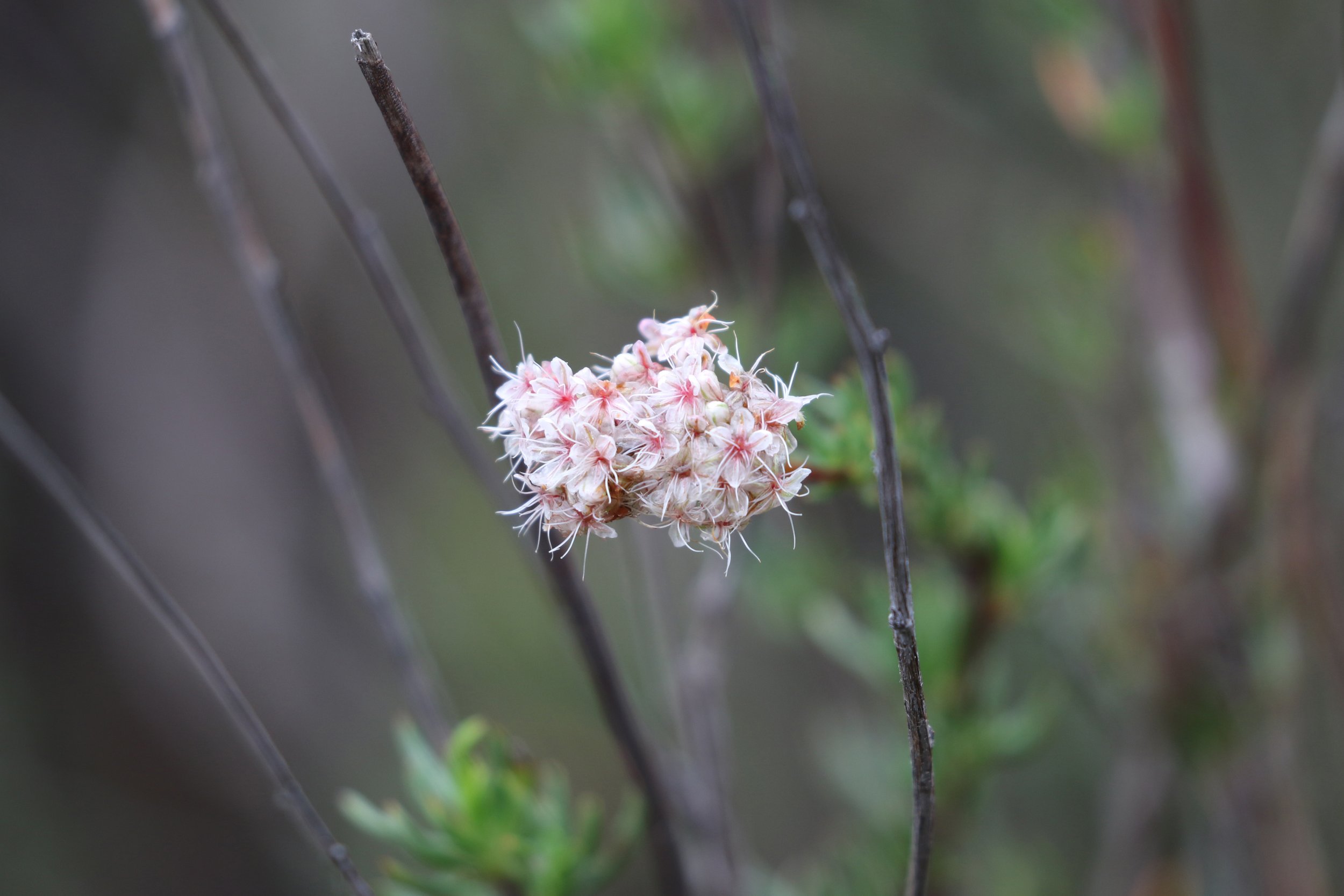This striking landscape photo, taken with a high-resolution camera, showcases a central flowering plant in exquisite detail. The photo is wider than it is tall, focusing sharply on a cluster of vibrant flowers. Each flower, adorned with pink centers and pointy white appendages that resemble narrow, white worms, stands in stark contrast against a blurred, foggy background. In total, about 20 flowers are captured, all emerging from a single branch. Two prominent brown stems rise through the middle of the frame, adding to the plant's intricate structure. Around the sharply-focused flowers, the background fades into obscurity, revealing hints of additional green foliage and branches, which blend into a misty, forest-like setting. The overall impression is one of serene natural beauty, isolated for artistic emphasis.